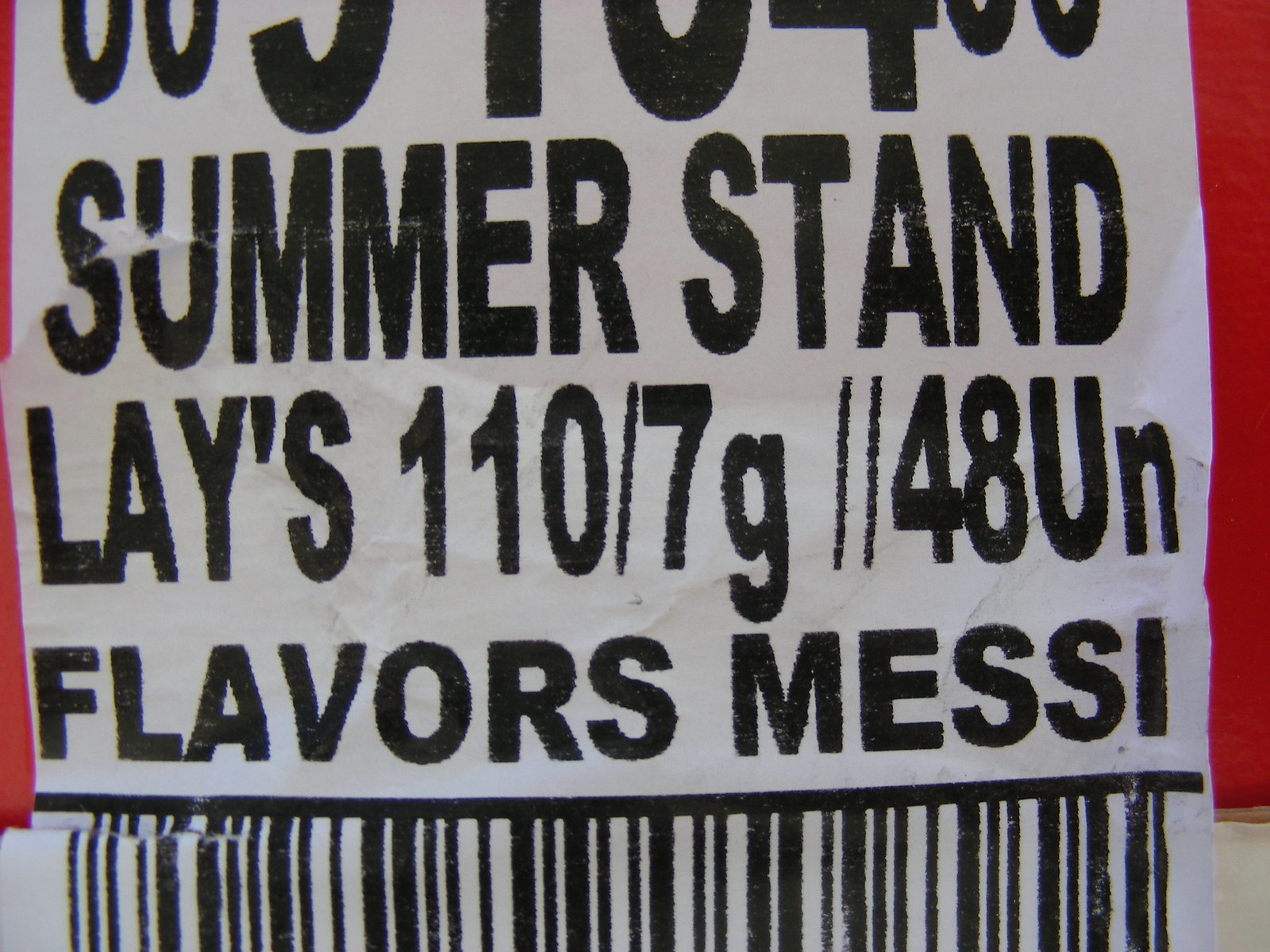This image captures a close-up of a label, possibly from packaging or a sign, set against a plain white background. The text, displayed in bold black font, reads: "SUMMER STAND LAYS 110/7G48UN FLAVORS." To the left and right edges, there are thin strips of red adding a touch of color contrast. The label also includes the word "MESSY" prominently spelled out as "M-E-S-S-I." Beneath this text, a horizontal black line runs across the label, followed by a barcode situated at the bottom, ensuring the item can be scanned for retail purposes.